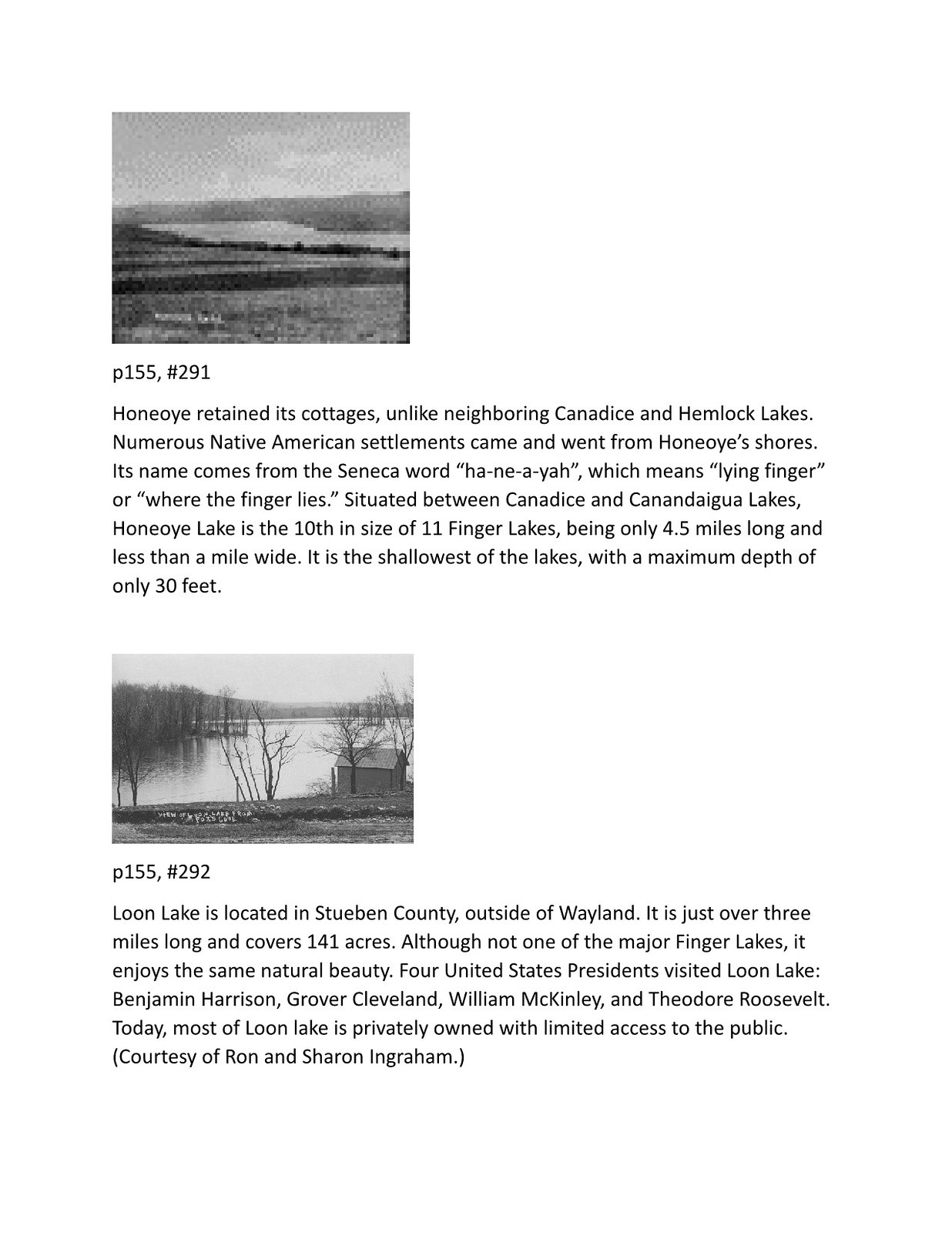The image consists of two small black and white photographs positioned on a white background, each with accompanying descriptive text below. The top photograph, labeled "P155, #291," appears to be a landscape that potentially features plains or a lake in the background, though details are faint. Beneath this image, a paragraph describes Honeoye Lake, emphasizing its retention of cottages unlike its neighboring lakes, Candace and Hemlock. It notes the numerous Native American settlements that historically occupied Honeoye's shores and explains that the name derives from the Seneca word "Haneayah," meaning "lying finger" or "where the finger lies." Situated between Candace and Canandaigua Lakes, Honeoye Lake is the tenth largest of the eleven Finger Lakes, measuring only 4.5 miles long and less than a mile wide. It is the shallowest among them, with a maximum depth of merely 30 feet.

The lower photograph, labeled "P155, #292," is somewhat clearer and features a lake with a small building nearby and trees without leaves in the background. The text beneath this image discusses Loon Lake, located in Steuben County near Wayland. It states that the lake spans just over 3 miles and covers 141 acres. Although not one of the major Finger Lakes, Loon Lake is noted for its natural beauty and historical significance, having been visited by four U.S. Presidents: Benjamin Harrison, Grover Cleveland, William McKinley, and Theodore Roosevelt. Presently, most of Loon Lake is privately owned with limited public access. This information is credited to Ryan and Sharon Ingram.